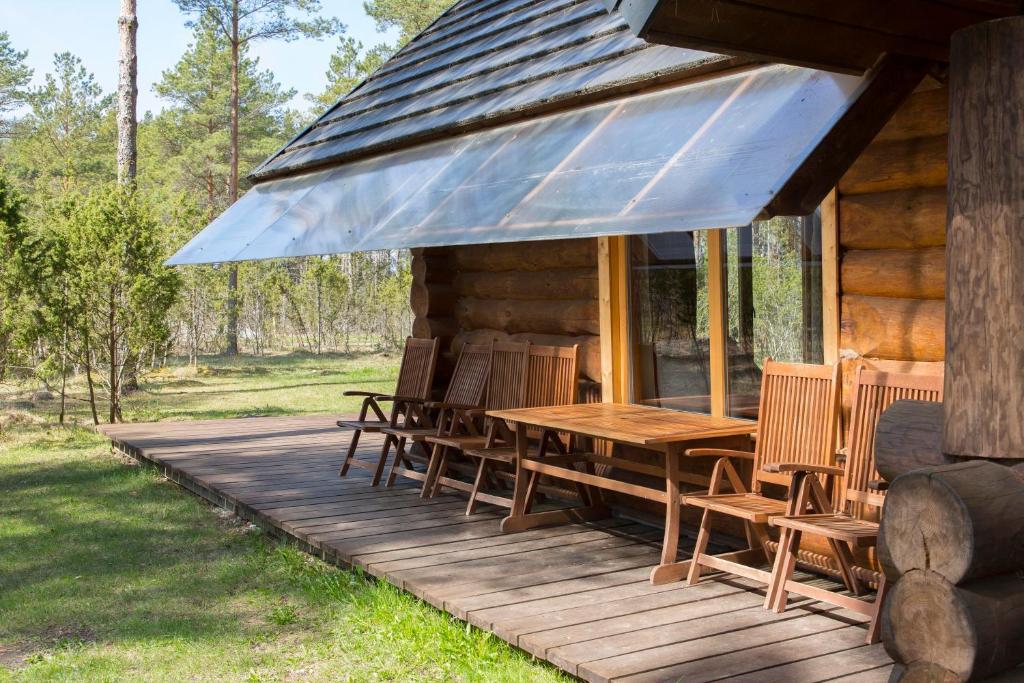The photograph captures a serene, sunny outdoor setting showcasing the side view of a log cabin. Positioned on the right side of the image, the cabin—constructed from variously shaded, weathered brown logs—features a slanted roof with an attached metallic-gray overhang that partially covers a spacious wooden deck. The deck, constructed from vertical off-gray planks, holds a large wooden table flanked by six tan brown wooden chairs, with two positioned in front of a pair of clean, white-framed windows. Green grass, interspersed with patches of brown and tan, extends from the cabin towards the left side of the image, transitioning into a field bordered by a variety of evergreen pine and fir trees of differing heights. The trunks of these trees, visible on the left portion of the photo, rise against a backdrop of a vivid blue sky.